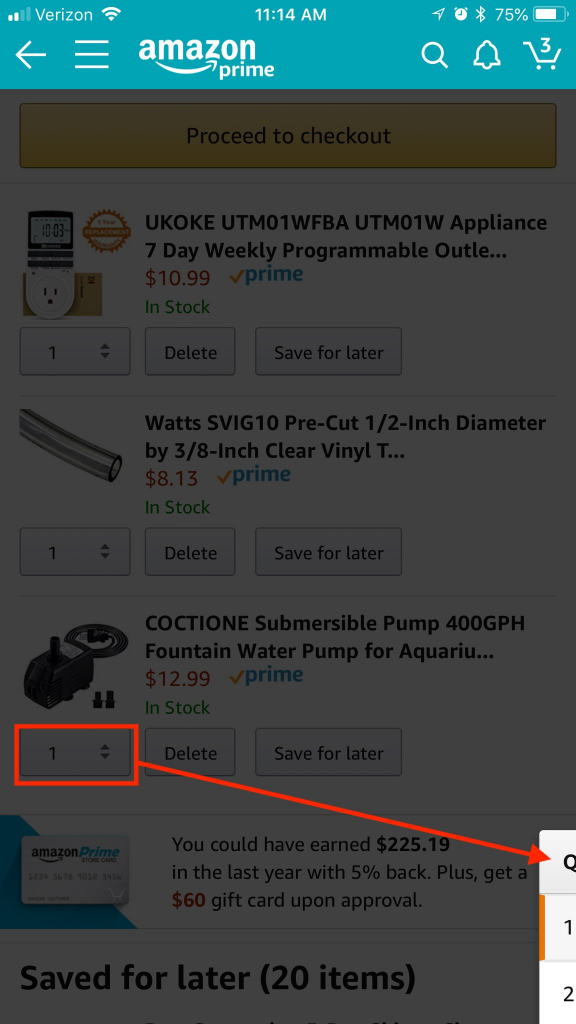This screenshot captures a webpage from a mobile device, specifically on a Verizon network with Wi-Fi enabled. At the top of the screenshot, there's a distinct blue banner with white text. The status bar reveals two bars of Verizon signal strength, the time displayed as 11:14 a.m., and a battery level of 75%. The cart icon indicates that there are three items currently in the shopping cart.

Beneath the status bar, the webpage content is somewhat grayed out, making it difficult to discern. However, the top section is labeled "Proceed to Checkout." The first item listed is the "Yukoke UTM01 WFBA UTM01W Appliance," described as a 7-day weekly programmable device. The item is priced at $10.99, marked in red text, accompanied by a check mark and the blue "Prime" label, indicating that it is eligible for Amazon Prime and in stock. Below this product, there is a section for adjusting the quantity, currently set to one, and options to either delete the item or save it for later.

The second item in the cart is a "Watts SPIG 10 pre-cut 1 1/2 inch diameter by 3 1/8 inch clear vinyl," priced at $8.13.